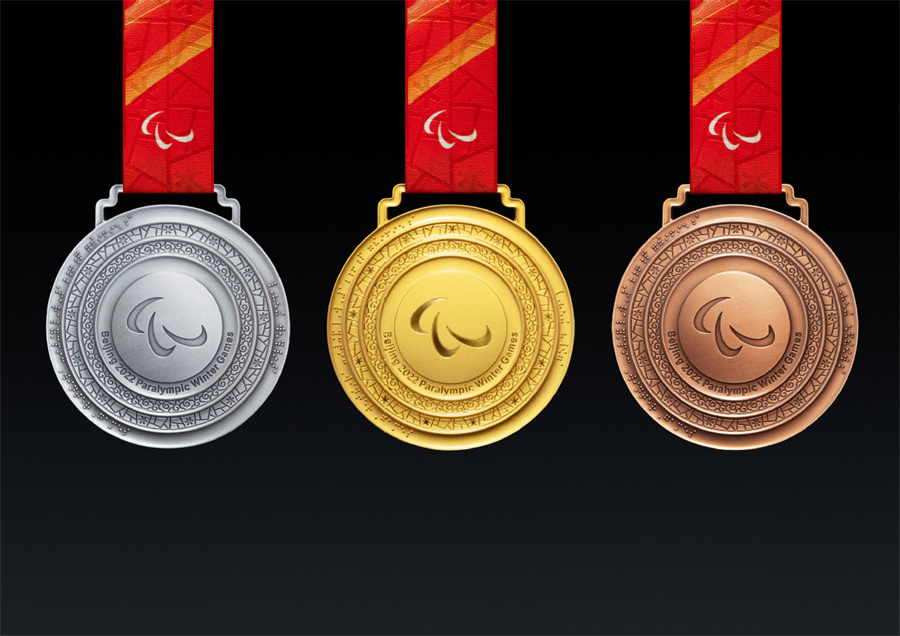This digitally created image features three medals prominently displayed against a solid black background. Each medal is suspended from a bright red ribbon adorned with diagonal orange and yellow stripes and embossed geometric patterns. The medals, aligned centrally and hanging to the halfway point of the image, are ordered with the silver medal on the left, the gold medal in the center, and the bronze medal on the right.

Each circular medal includes a series of concentric circles filled with distinctive patterns. The innermost circle showcases three white swoosh shapes, which are mirrored on the lanyards. Surrounding this, there are three thin rings and one prominent middle ring. The outermost ring includes braille inscriptions. At the bottom of the first circle outside the center, there is curved text that reads "Beijing 2022 Paralympic Winter Games."